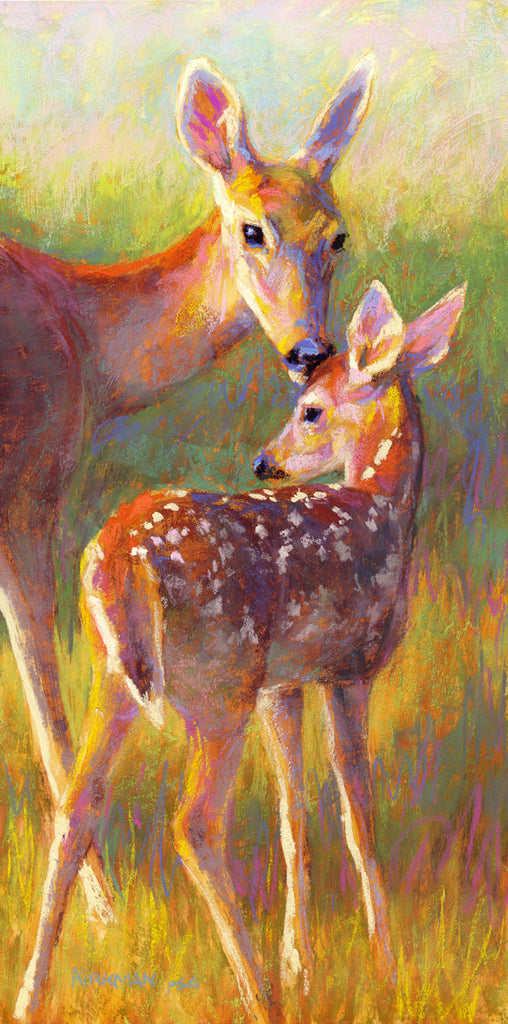This captivating watercolor painting by the artist Kirkman, whose signature appears in gray on the bottom left, depicts a serene and sunlit scene involving a doe and her fawn in a tall, grassy area. The golden grass in the foreground transitions to green foliage in the background, suggesting a natural, vibrant setting on a sunny day. The doe, slightly cropped and appearing from the left side, lovingly licks the head of her fawn, which stands small yet prominently with distinctive white speckles on its brownish-yellow coat. The fawn, facing the right but looking left, mirrors the tender connection with its mother. Their shadows are softly cast on the golden grass, enhancing the depth and warmth of the scene. Bright, expressive light colors dominate the painting, enriching the detailed portrayal of this intimate wildlife moment.